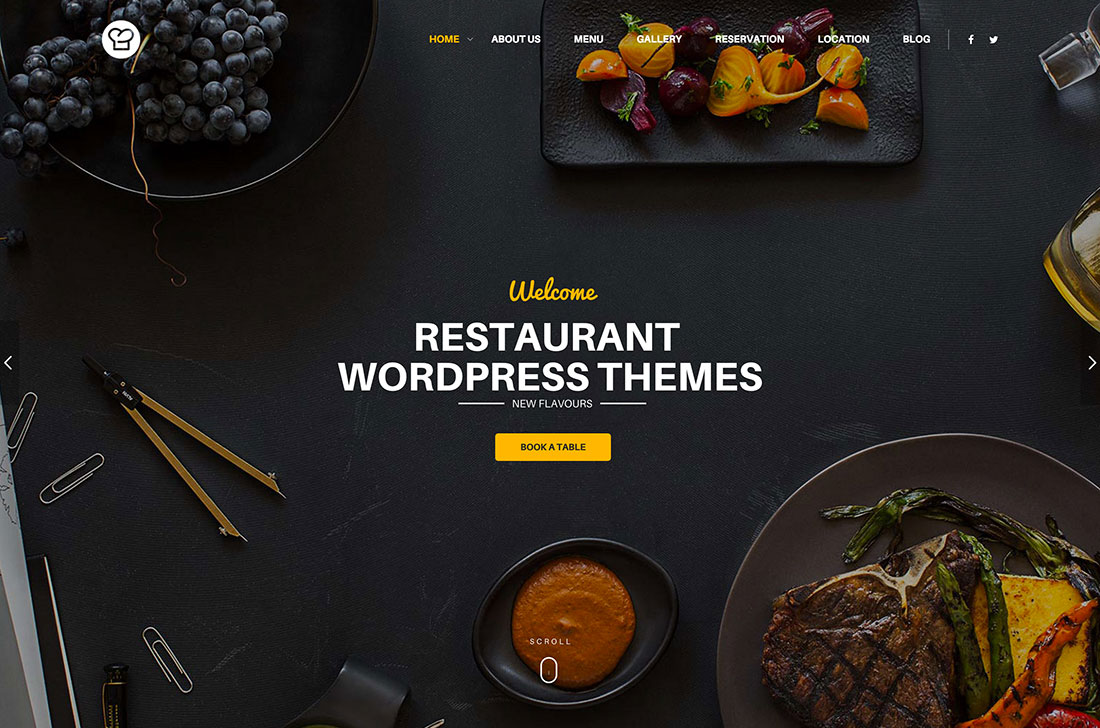In the top left corner, a chef's hat is displayed within a white circle. The website's navigation includes sections such as Home, About Us, Menu, Reservation, Gallery, Location, Blog, and Welcome, all highlighted in yellow, except for "new flavors" which is in white. There is a yellow square icon for booking a table. 

The central image features a diverse spread: a metal compass is used for drawing circles, three paper clips, a pointed rod, and a magnifying glass are scattered over white paper. A platter of grapes sits nearby. 

The main dish consists of a steak accompanied by sweet potatoes and overly burnt asparagus. Beside it, a slice of burnt cheese is visible. Another square white plate holds orange and purple beets garnished with what appears to be thyme. An ashtray is positioned in the top right corner, alongside a bottle of cooking oil.